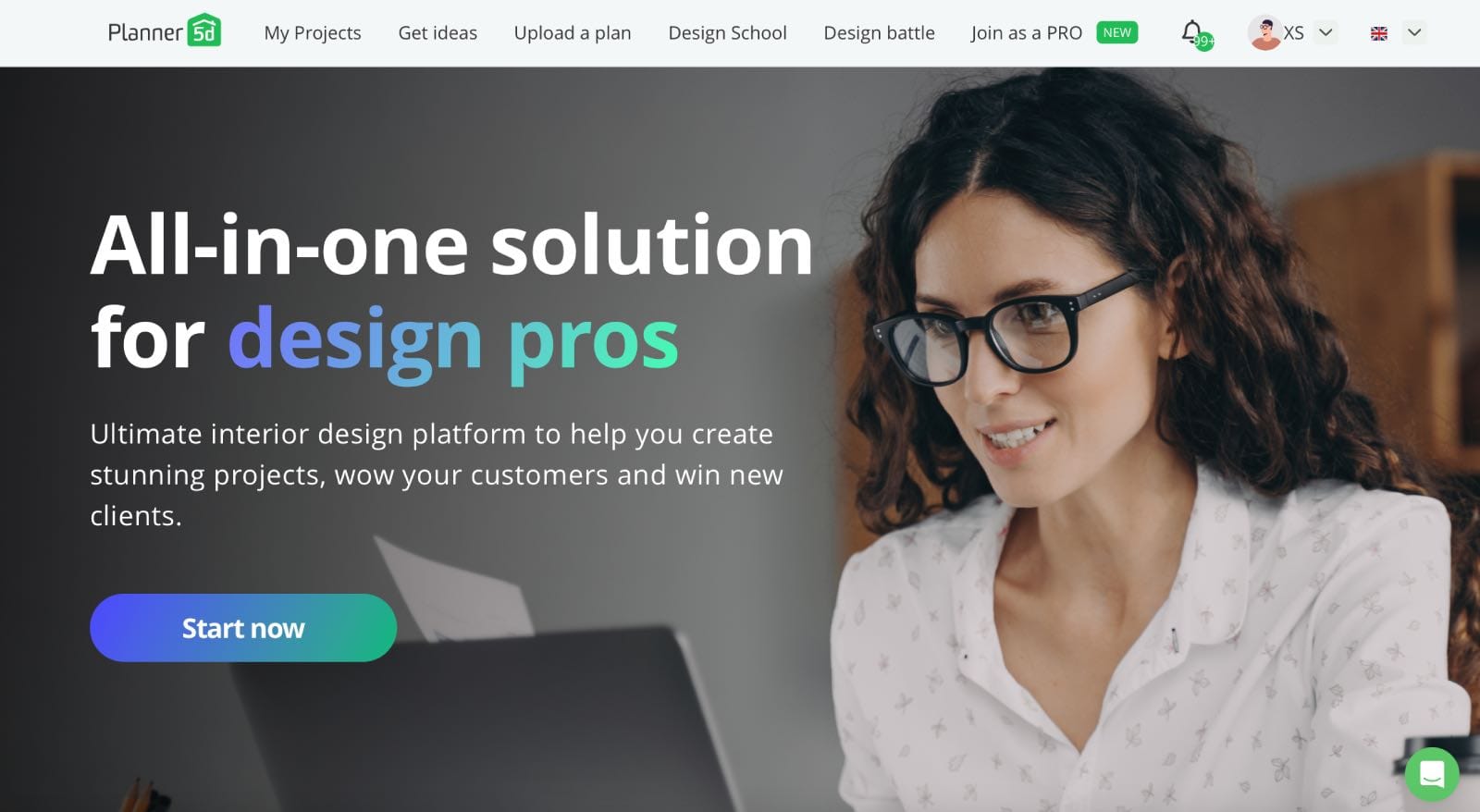This image features a page from the website Planner 5D, prominently displaying their logo, which resembles a house with a green interior and a stylized "5D" below a roof. The top of the page has a gray banner with several tabs: "My Projects," "Get Ideas," "Upload a Plan," "Design School," "Design Battle," "Join as a Pro," and a green button labeled "New." Additionally, there is a notifications icon indicating "19+" unread notifications, and a user profile icon marked with "XS" beside a dropdown arrow. To the right of these icons is the flag of Great Britain with another dropdown arrow.

The main image shows a young woman in her 30s, with dark brown hair highlighted with light brown streaks. She is wearing black-framed glasses and a light-colored blouse with an indistinguishable design, and she is smiling while looking at a laptop screen. The setting appears to be an office or a home office.

Accompanying text promotes Planner 5D as the "all-in-one solution for design pros," describing it as the "ultimate interior design platform to help you create stunning projects, wow your customers, and win new clients." Below this text is a button that transitions from blue to green, with white text that says "Start Now." At the bottom right of the screen, a green and white chatbot icon is visible.